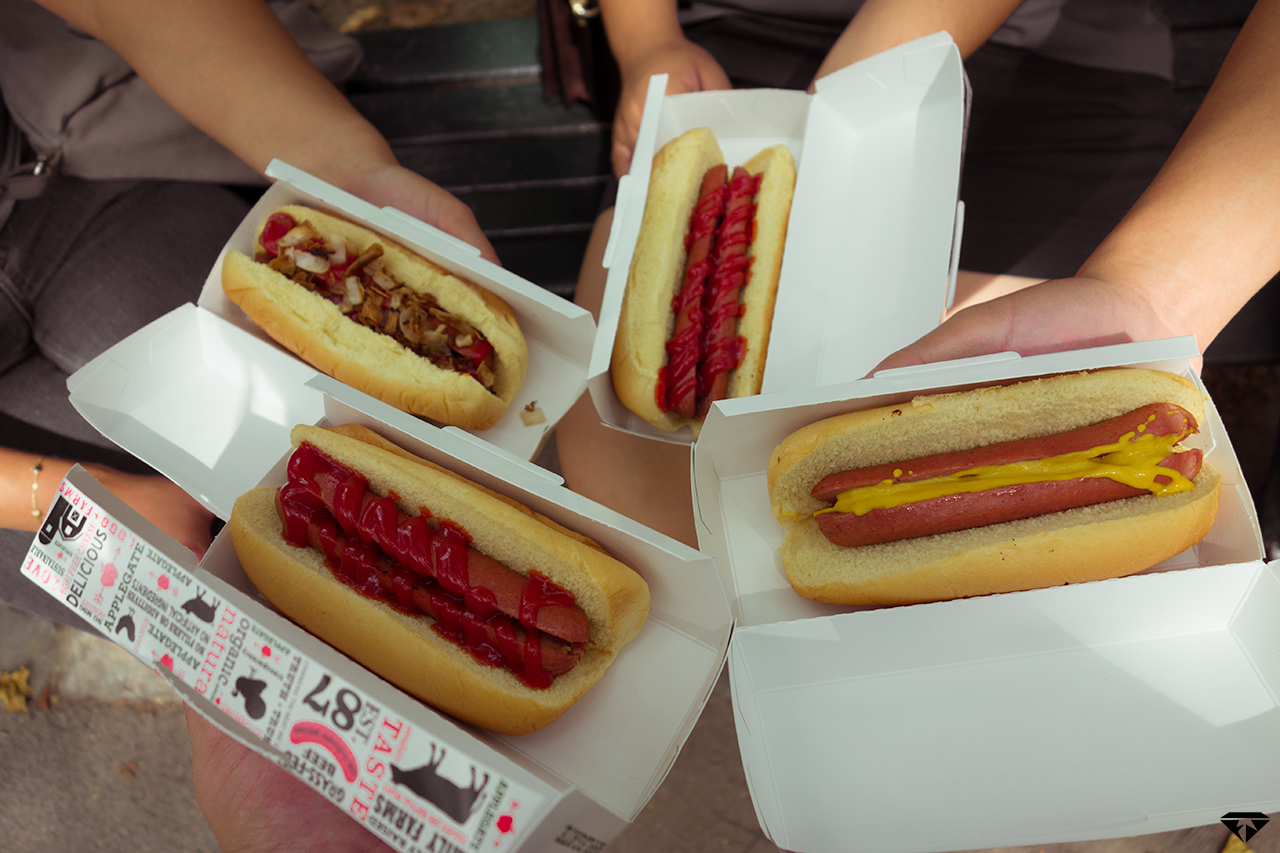In the image, three to four people are holding out four hot dogs, each nestled in white cardboard containers. The individuals seem to be sitting in a circle, collectively showcasing their food. Each hot dog is cut in half lengthwise, with various condiments adorning them. The hot dog on the far left has a red hot dog nestled in a brown bun, topped with red sauce, possibly ketchup. The second hot dog features a more elaborate array of toppings including what looks like mushrooms, onions, and additional sauces. The third hot dog is simpler, with just ketchup, while the fourth one sports only yellow mustard. The cardboard box of the first hot dog displays a design with intricate details: "Taste," "Established 87", a black cow, a red hot dog, various farm animals like cows, pigs, and chickens, a barn, and the words "delicious," "grass-fed beef," "organic," and "natural" emblazoned across it. The photograph captures the collective enthusiasm and anticipation of enjoying a meal together.